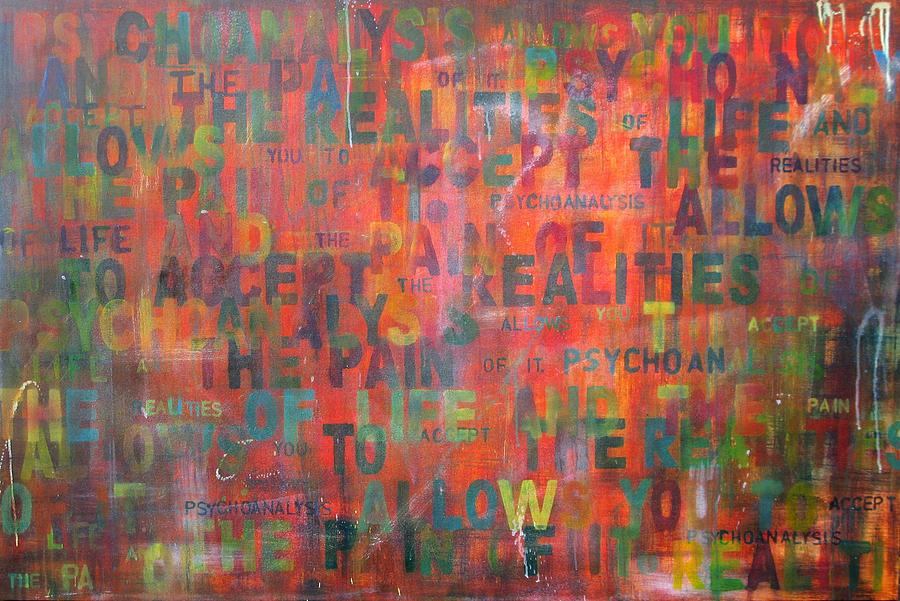This rectangular artwork, wider than it is tall, features an eye-catching mural characterized by an intricate overlay of spray-painted words on a vivid orange-red background. The piece captures a fusion of emotions and philosophical insights through its text, which includes phrases like "accept the realities," "the pain of psychoanalysis allows life," "realities of life," and "love." These words, often repeated and intertwined, are rendered in a vibrant palette of green, blue, dark red, light blue, light green, yellow, and occasionally black. The block letters are strategically placed, creating a chaotic yet harmonious visual symphony. The mural serves as a powerful statement, blending colorful aesthetics with profound thematic elements.